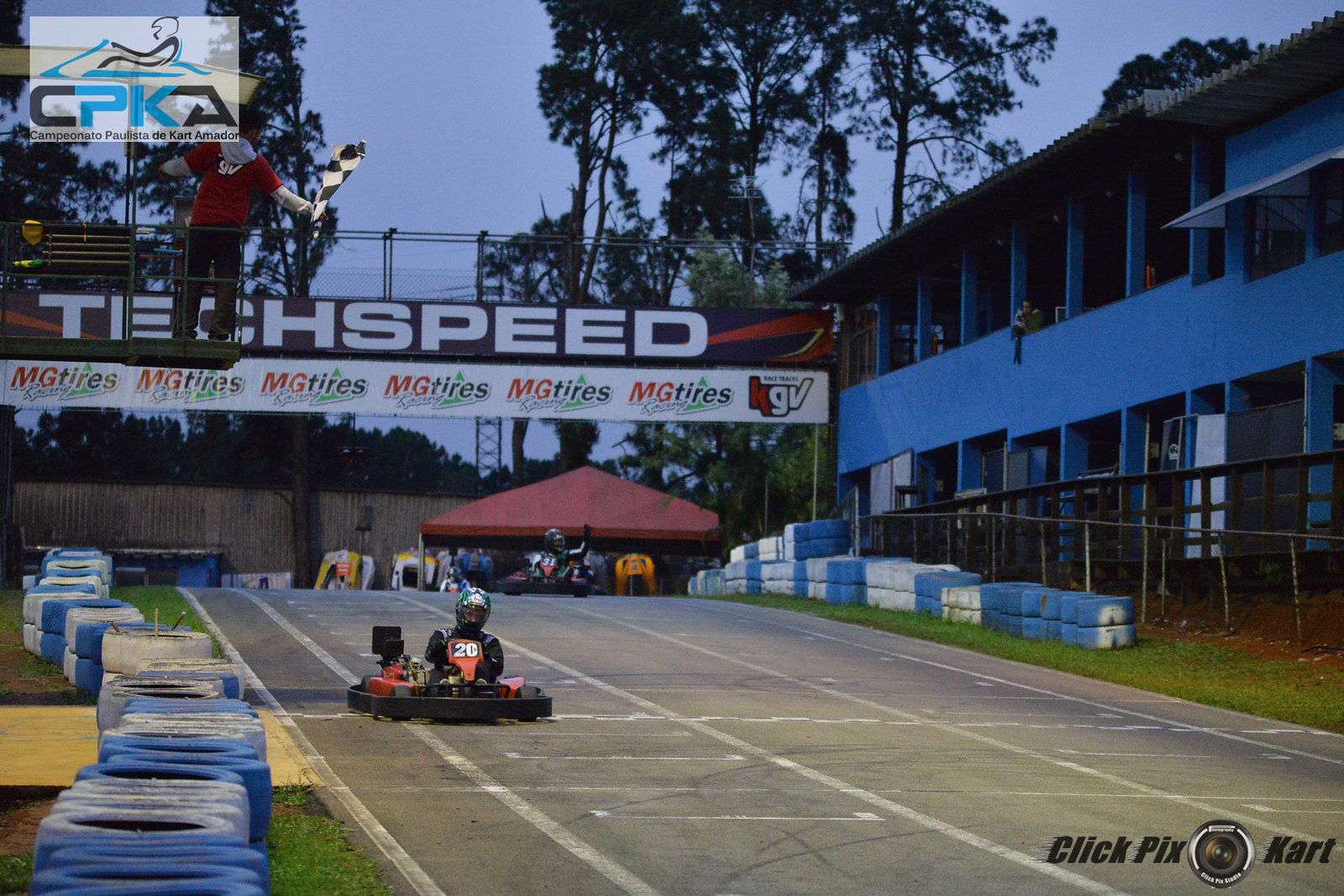This photograph captures a twilight scene at a go-kart race, with the sky exhibiting a darker, light blue hue indicative of the setting sun. The track is divided into three main lanes with an additional smaller lane on the side. In the foreground, a single go-kart, orange and black in color, driven by a racer wearing a green helmet and a black outfit, is prominently featured with the number 20 visible on their chest. A person dressed in a red shirt and black pants stands elevated on a metal walkway above the track, energetically waving a black and white checkered flag.

To the right, dark green trees further enhance the twilight ambiance. Additionally, a light blue structure, possibly a pavilion or building, can be seen. The upper side of the image features a banner with white "TechSpeed" lettering against a black background and an orange design, positioned right underneath another banner stating "MG Tires." Near the bottom right edge, the words "Click Pics Kart" with a 'K' are visible. The entire scene encapsulates the thrilling moment right before the end of the race, while another go-kart, slightly trailing behind, is part of the action.